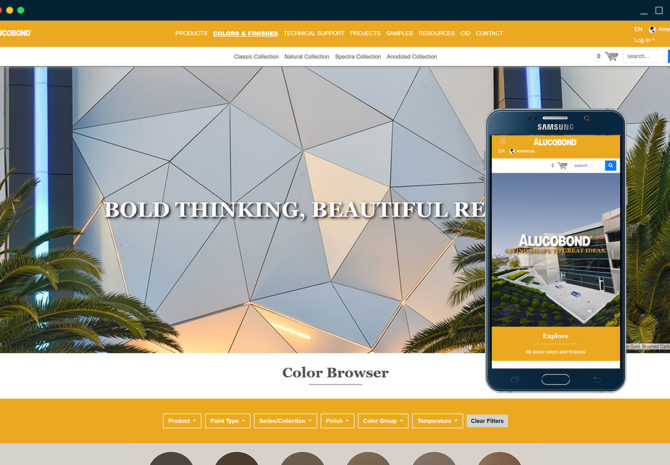The image is a horizontally rectangular screenshot taken from a website, although the left and right edges of the frame appear to be cut off. The website belongs to a company named "Beluco Bond." At the top of the page, there is a deep orange horizontal banner containing navigational options, including "Products," "Colors and Finishes," "Technical Support," "Projects," "Samples," "Resources," and "Contact." The "Colors and Finishes" option stands out as it is both bolded and underlined. 

Directly below the banner, the page presents further choices categorized into different collections: "Classic Collection," "Natural Collection," "Spectra Collection," and "Anodized Collection." The text here appears smaller and is somewhat difficult to read.

The central part of the image features a background that appears to show a glass building facade. The glass sections are designed in an angled, triangular pattern. Overlaying this background, in white text, are the words "Bold Thinking, Beautiful." Further down, the page features an option labeled "Color Browser." 

The overall impression of the webpage suggests a focus on architectural materials, emphasizing aesthetic diversity and modernity in their product offerings.